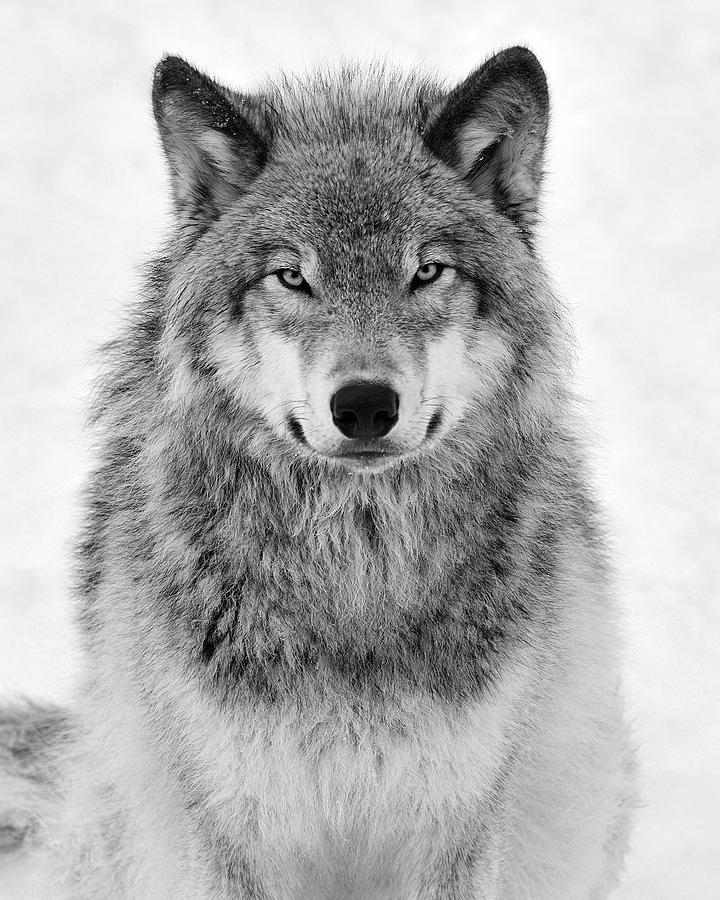This is a detailed black and white photograph of a majestic gray wolf set against a sky with patches of blue visible through a smattering of white clouds. The wolf, possibly male, is sitting on its haunches and staring directly into the camera with piercing light blue eyes that exude both intensity and a touch of gentleness. The wolf's ears are erect, showcasing black tips with lighter fur inside, and between them, tuffs of hair stand upright. He has a distinctive black nose, and his mouth forms a subtle, almost smile-like expression, adding a sense of calm to his powerful gaze.

The fur around his neck is darker, transitioning into a lighter shade as it moves down his body, becoming predominantly white lower down. His physique is captured in a pose that emphasizes his elegant structure, with hints of darker fur visible between his legs, on his haunches, and at the tip of his tail. Each strand of fur appears meticulously detailed, with shorter, smoother fur around his eyes contributing to his striking appearance. This captivating image not only captures the beauty and strength of the wolf but also evokes a sense of the wild and untamed.